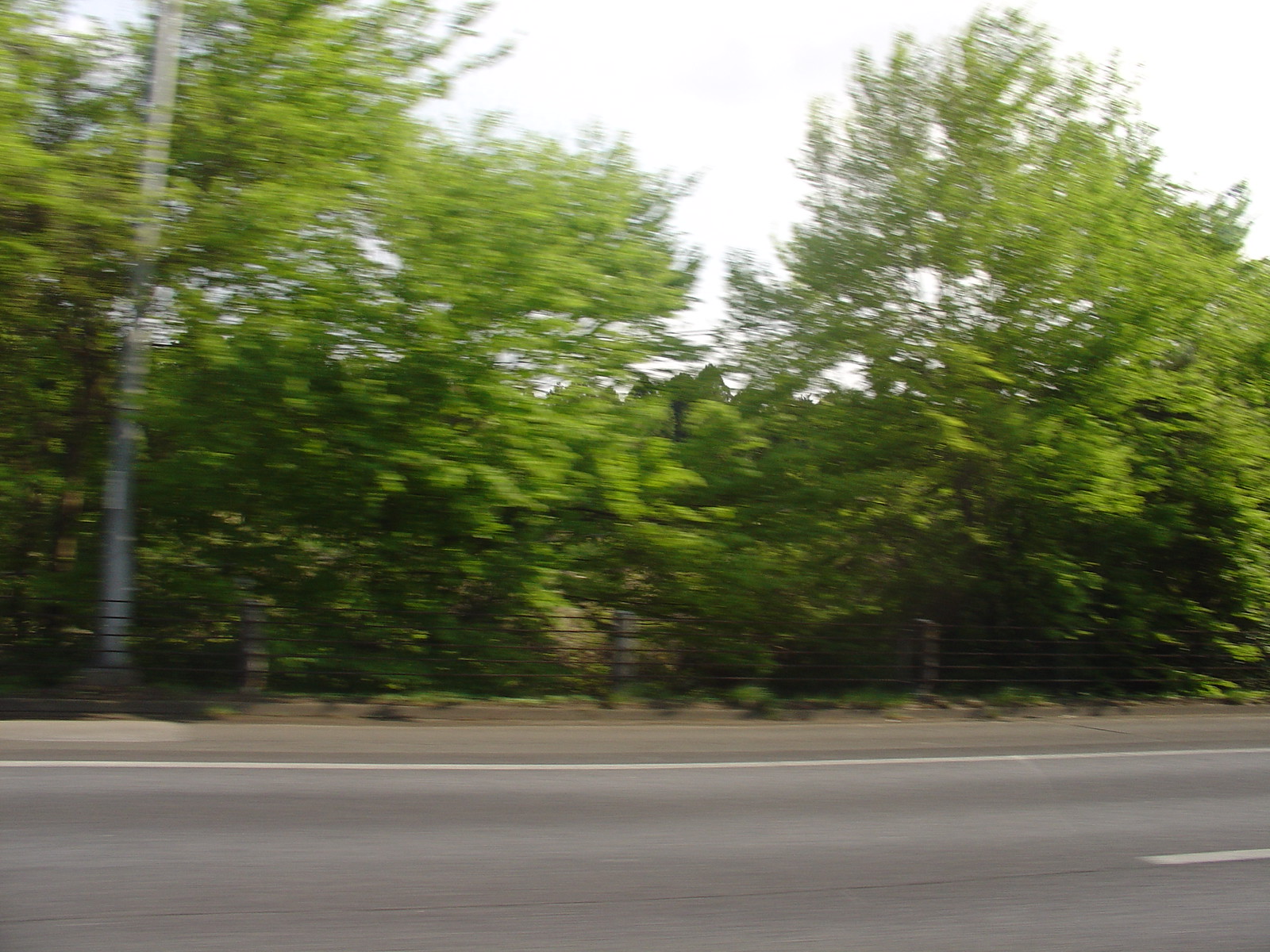This slightly blurry photograph captures a serene two-way street in a rural area. The asphalt road features white dashed lines down the center and solid white lines along the edges, emphasizing its structure. Notably, there are no cars present, adding to the peaceful atmosphere of the scene. On the far side of the street, a narrow sidewalk is visible, bordered by abundant trees, foliage, and brush. Peeping through the dense vegetation is a glimpse of a metal fence, suggesting a boundary or property line. The sky above is a very light, almost white, further enhancing the tranquil, almost ethereal quality of this rural landscape.